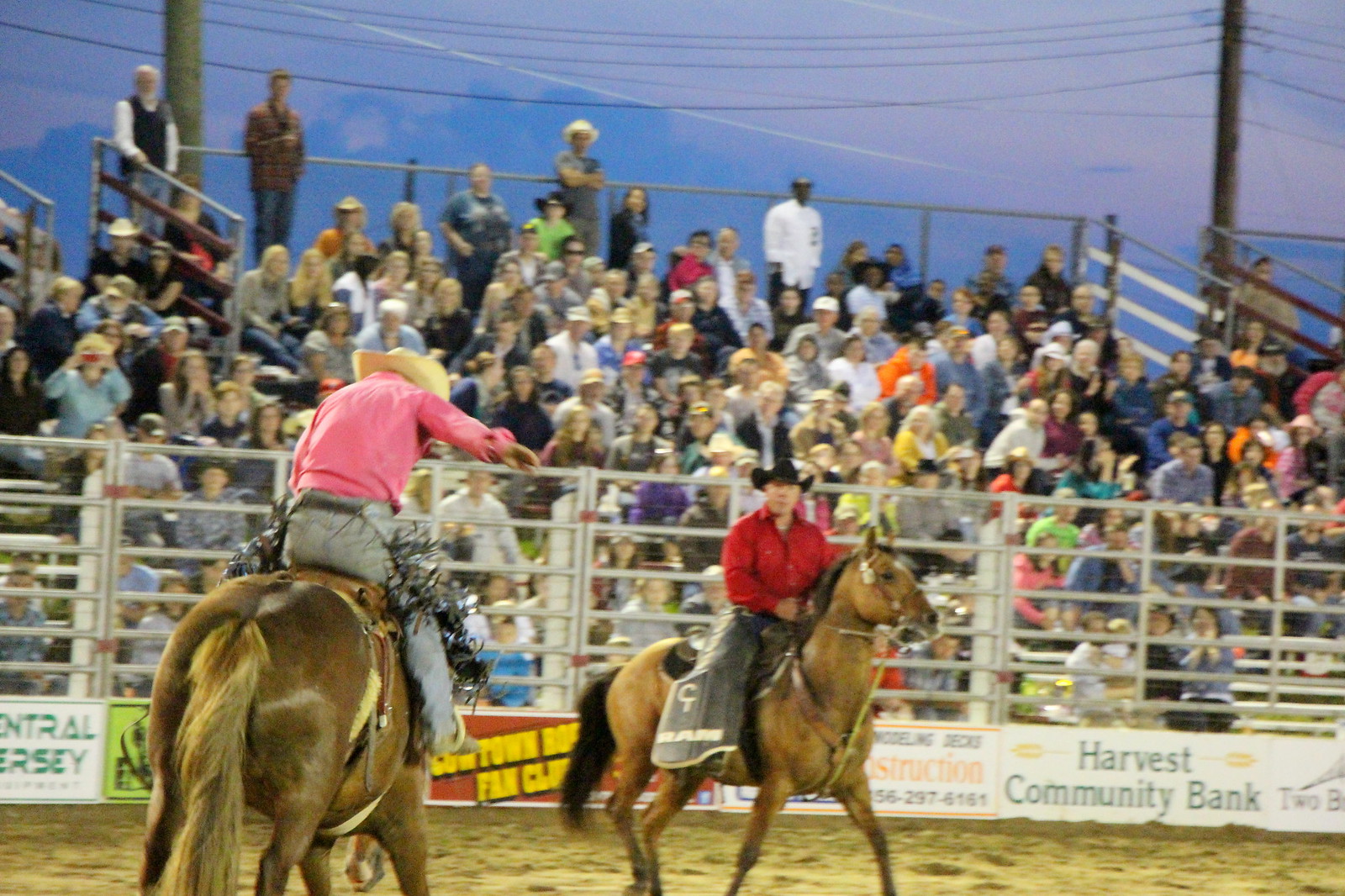This dynamic photograph captures an intense moment at an outdoor rodeo. The dirt arena, enclosed by fencing adorned with logos such as Winsor & Newton and Harvest Community Bank, is the central focus. In the background, bleachers packed with spectators rise about 15 rows high, enveloped by a landscape of majestic mountains, under a sky tinged with the hues of sunset.

At the heart of the action, two cowboys command the scene atop their brown horses. The cowboy in the foreground, wearing a pink t-shirt, light jeans, and a tan cowboy hat, is riding one-handed as his horse bucks wildly, captured mid-motion. This horse has a dark body complemented by a blonde mane and tail. Nearby, in the middle of the arena, the second cowboy, sporting a long-sleeve red shirt, dark pants, and a black cowboy hat, steadies his slightly lighter-colored horse with both hands, as it trots along calmly. Both riders are intently in action amidst the dusty commotion, with the audience eagerly watching behind a metal barrier designed for optimal viewing. The rich details of movement, atmosphere, and the anticipation in the crowd beautifully encapsulate the spirit of the rodeo.